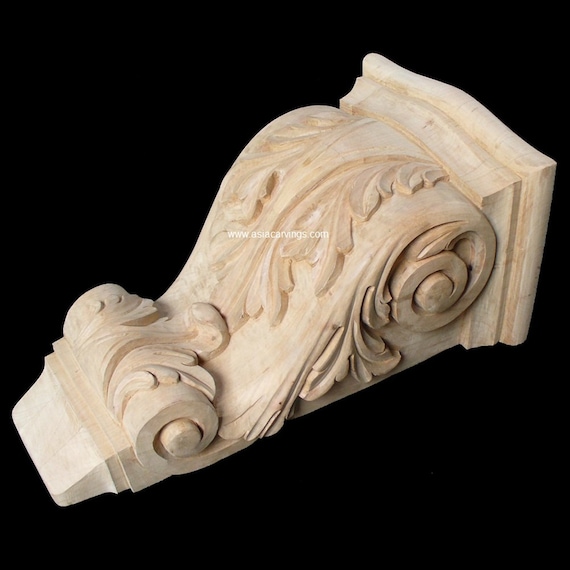This image shows a decorative wooden sconce holder, designed to be affixed to a wall. The piece tapers elegantly from a narrow base to a wider top, and features intricate carvings resembling a fleur-de-lis and foliage patterns. The decorative motifs lend it a Greek or classical architectural aesthetic. The top of the sconce flares out to form a small shelf, suitable for holding a candle, small plant, or other decorative items. While it has a stone-like appearance at first glance, it is actually made of wood, and a plastic sleeve is seen at the base, possibly to prevent splitting. This sconce could be used to frame a centerpiece, placed on either side of a fireplace, or as an ornamental accent in a doorway. The image itself has a black background with a watermark at the center that reads "www.asiacarvings.com."